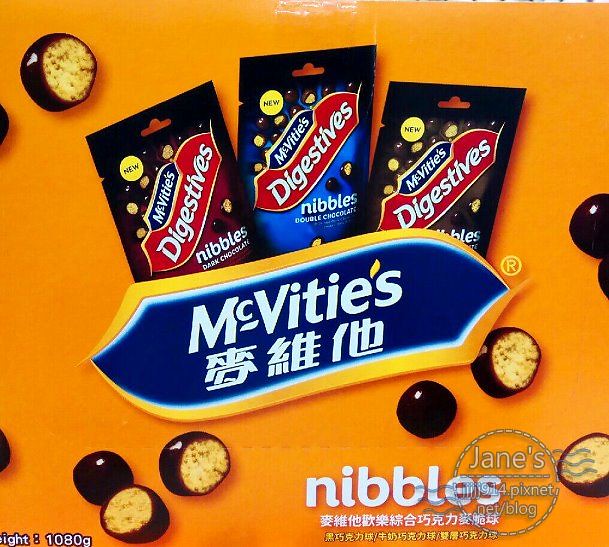The advertisement showcases three varieties of McVitie's Digestives Nibbles, each in distinctively colored packaging displayed against a warm yellow background. The three bags, arranged at slight angles away from each other, highlight the different flavors: one with dark chocolate in a black package featuring red and blue accents, one labeled as double chocolate, and a third, whose variety is indistinguishable. Each package prominently displays the McVitie's name with the text "Nibbles" in white on a red background. To the left of each package, a yellow circle announces the "new" status of the product. Scattered around the photo are enlarged images of the actual candies, both whole and halved, revealing their chocolate exteriors and textured wafer-like insides. At the very bottom, the word "Nibbles" is again noted in white text, accompanied by additional characters presumed to be in a foreign language, possibly Chinese, which are also found beneath the main McVitie's text in the center of the image. The combination of vibrant colors, clear product depiction, and detailed representations of the candies makes this advertisement visually compelling.